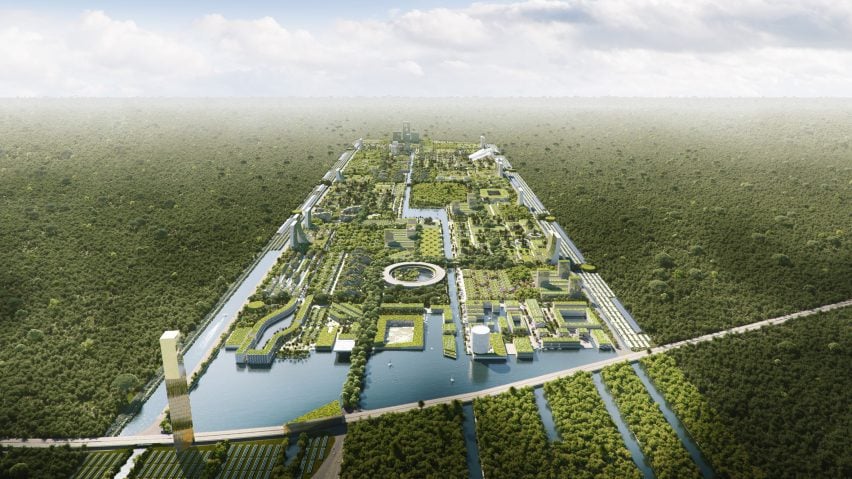The image, an aerial photograph or possibly a computer-generated rendering, showcases a meticulously manicured green space that forms a central rectangular area, reminiscent of a city or a sophisticated layout. The foreground of this central area is characterized by an array of still bodies of water, reflecting the surrounding environment and bordered by lush greenery. There is a distinctive, curving white road made of concrete that cuts through the well-kept expanse. Within this manicured rectangle, various types of structures are visible, including square buildings, round towers, and areas that might be water treatment facilities, all interspersed with greenery.

The edges of the image transition into dense, ungroomed woodlands with trees packed closely together. At the very top of the image, the horizon is marked by a light blue sky and numerous fluffy, white clouds, creating a foggy effect over the distant tree areas. A portion of the sky in the upper left-hand corner reveals a clearer blue hue. The significant use of green dominates the landscape, punctuated by the occasional concrete road and water reflections, adding to the serene yet structured aesthetic.